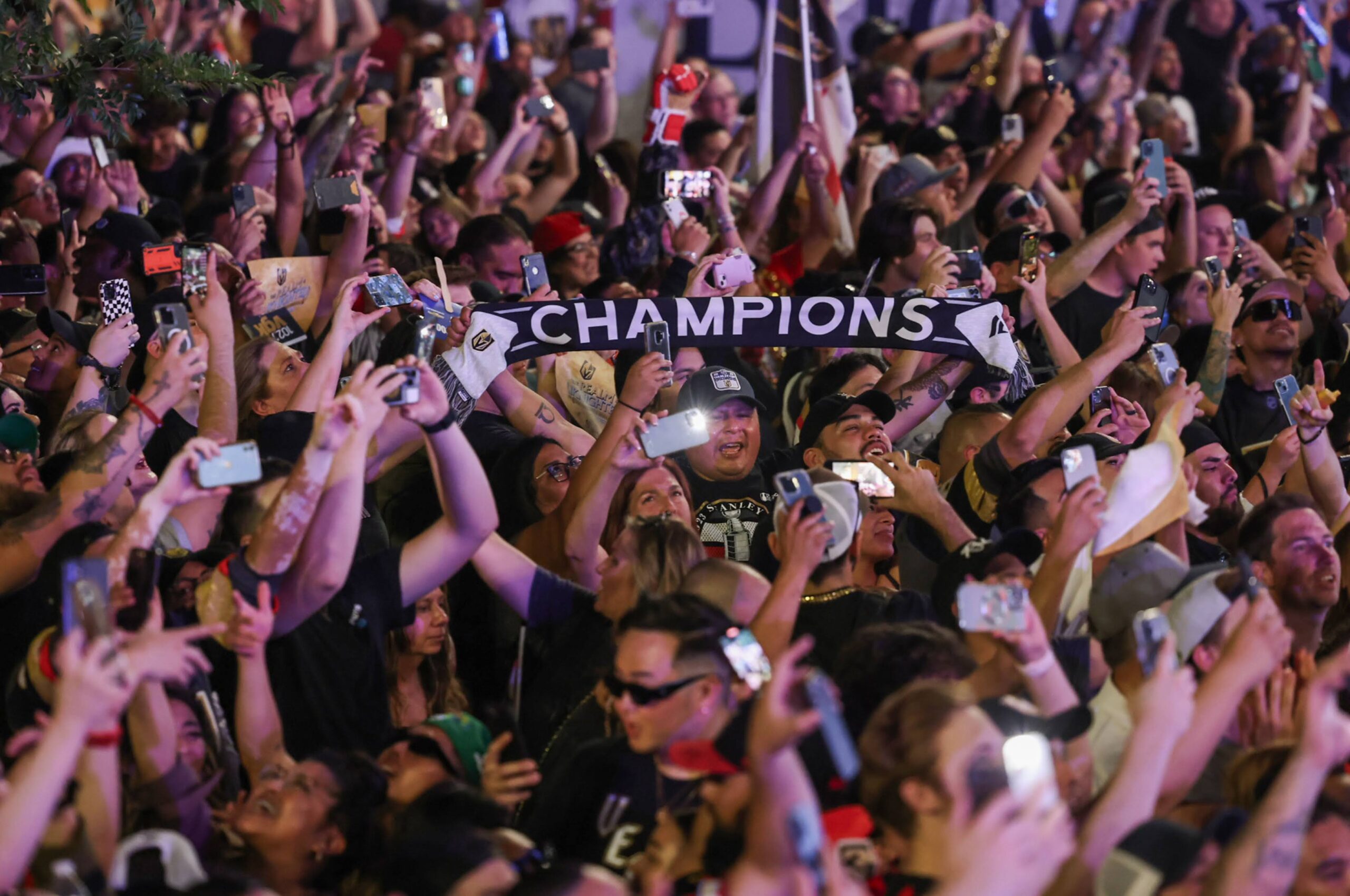This color photograph captures a festively packed crowd of enthusiastic people celebrating, likely at a concert or similar event. The image is taken from a slightly elevated angle, showing a diverse group of men and women, primarily younger to middle-aged, standing close together on a floor with no visible seating behind them. Many individuals in the crowd are holding up their phones, some with flashes on, to record the joyous moment. Hands are raised in the air, with one person notably pointing a finger upwards. 

The crowd is diverse, with a notable Asian man wearing black sunglasses and sporting a stylish haircut among primarily Caucasian attendees. Many of the men are wearing baseball hats. At the center of the image, two people are proudly displaying a black and white banner with the word "Champions" boldly printed across it. In the background, a flag-like object is visible, and a wall with what appears to be an exit door can be seen. The crowd extends throughout the frame, their hands and devices contributing to a dynamic and lively atmosphere.